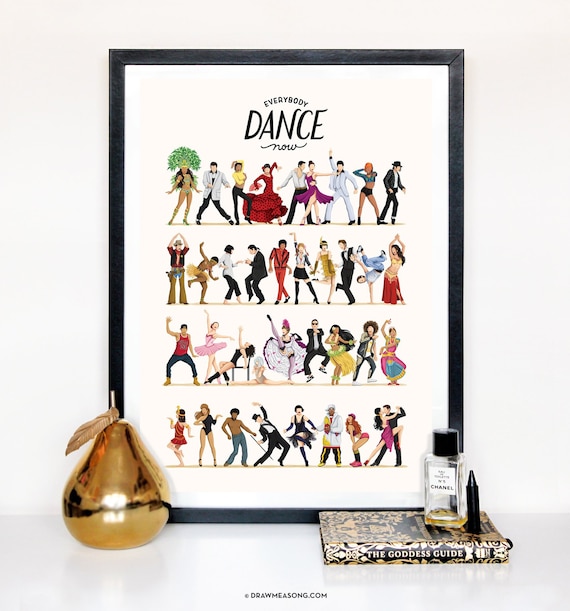The image features a meticulously arranged tablescape centered around a framed print with a bold heading that reads "Everybody Dance Now!" The print showcases four rows of various iconic dancers from different movies and eras, including notable figures like John Travolta from "Saturday Night Fever" and "Pulp Fiction," Michael Jackson, and dancers from "YMCA." The backdrop is a crisp white wall, enhancing the vibrant and diverse cartoon-style dancers depicted in the print. Positioned against the white background, the thin black-wooden frame elegantly encloses the artwork, adding a touch of sophistication.

In the foreground, a gold pear statuette commands attention on the left. To the right, there's a book titled "The Goddess Guide" placed horizontally, atop of which rests an almost empty bottle of Chanel No. 5 perfume and a black marker-style pen. This thoughtful arrangement of elements highlights a blend of luxurious and whimsical touches, creating a visually engaging and detailed display.